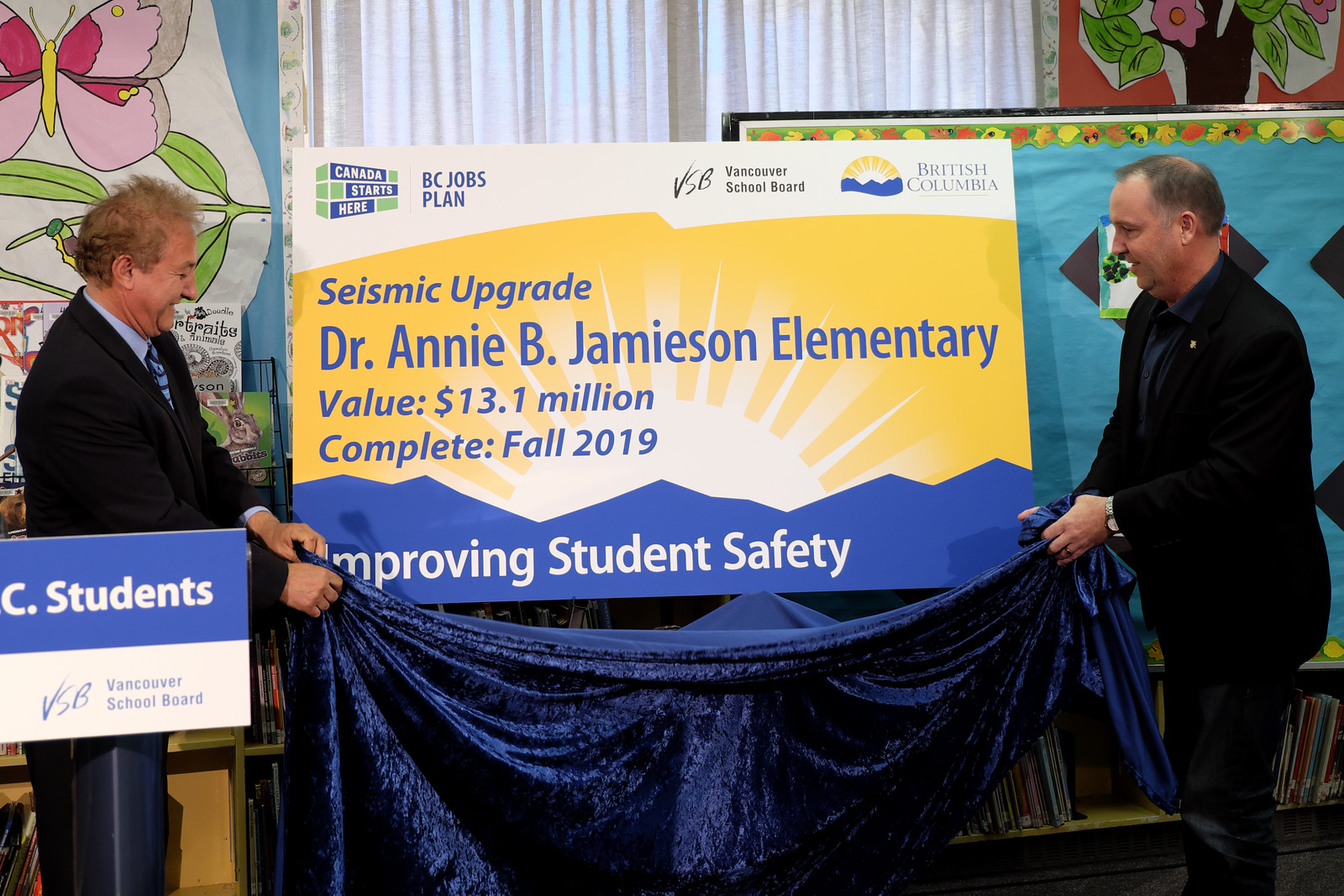In the photo, a significant moment is captured as two gentlemen unveil a large, colorful sign in what appears to be a school library adorned with white curtains and windows in the background. Both men, white males, are standing on either side of the sign, holding a blue velvet curtain that they have just pulled down. The man on the left is wearing a dark suit, a blue shirt, and a blue tie, with short brown hair and noticeable balding. The man on the right, also in a dark suit but with a dark shirt and tie, has short black hair and a bald spot. They both smile warmly at the sign they have revealed, which announces a "Seismic Upgrade Dr. Annie B. Jamieson Elementary" project valued at 13.1 million dollars and slated for completion in fall 2019. The sign is divided into three sections: the top part is white, the middle is yellow with a sunburst pattern and project details, and the bottom is blue with the phrase "improving student safety." The setting hints at a celebratory unveiling event, possibly marking the dedication of the upgrade, with a podium labeled "Vancouver School Board" and a shelf filled with books visible in the background. On either side of the image, colorful signs add to the festive atmosphere.